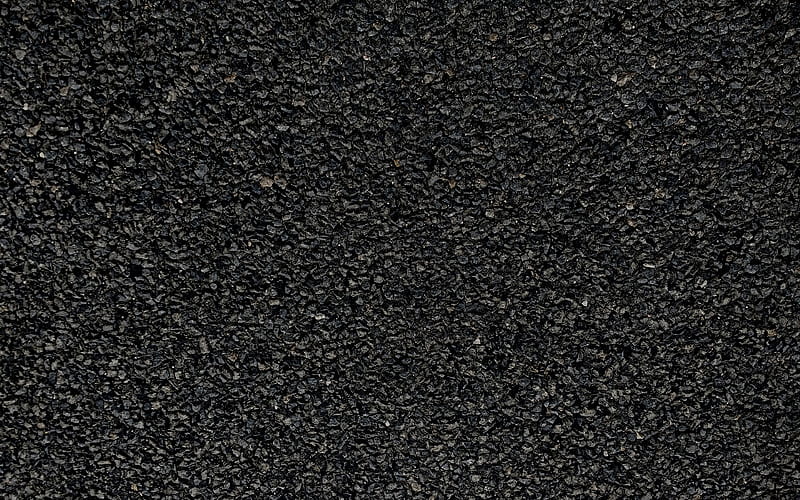This image features an extreme close-up photograph of what appears to be freshly poured black asphalt, filling the entire frame from edge to edge. The texture is highly detailed, showcasing the tiny, mixed aggregates that make up the surface. Scattered throughout the predominantly black and gray surface are minor flecks of brown and white, adding subtle contrast. The high magnification focus allows us to see the intricate divots and individual granules within the asphalt, giving the appearance of a textured, almost organic landscape. There are no other objects or disturbances present in the image, emphasizing the pure, unstepped surface of the asphalt.